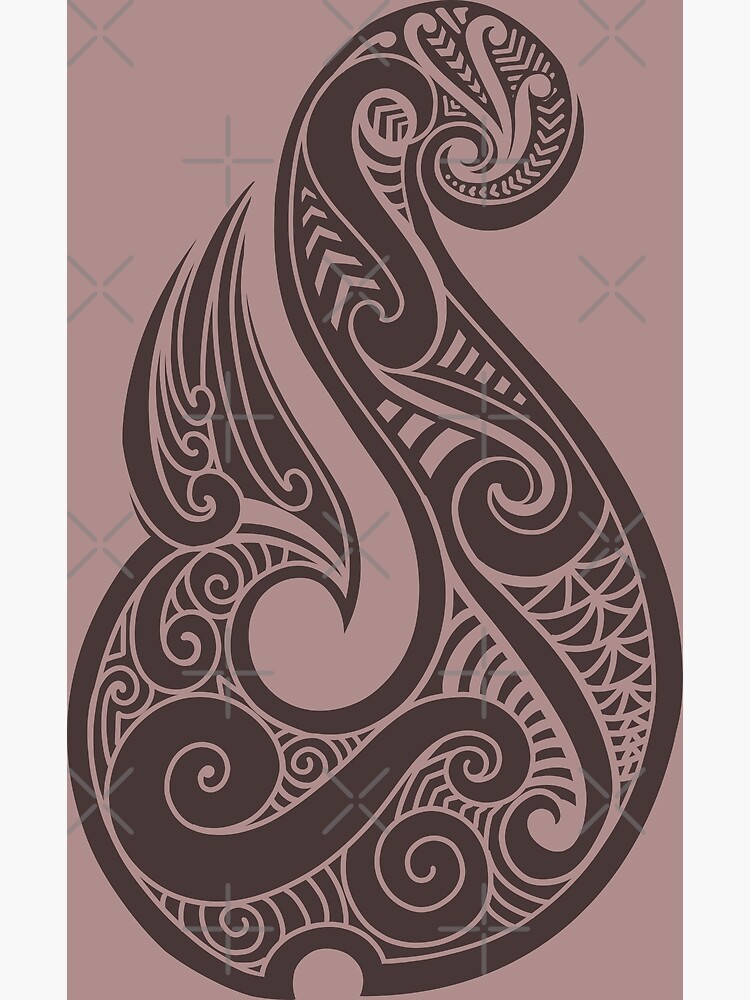The image features a highly detailed symbol against a grayish-plum background. Dominating the image is a large, ornate, black, S-shaped figure, reminiscent of both a dragon and a swan with intricate scrolled detailing. The upper part of the figure is tightly curled with a smaller loop, while the lower part expands into a broader, more pronounced curve. The inside of this S-shaped figure is filled with a complex array of black and white paisley patterns, swirling lines, and arrow-like designs. Additionally, there are smaller S-shaped figures within the larger one, including a brown one with a tan perimeter and another with a snail-like spiral, evoking the form of a circular staircase. Notably, the background hosts a subtle pattern of crosses and X's, adding depth to the overall design. The bottom tip of the symbol features an additional element, possibly resembling a wing, spike, or flame, further enhancing its elaborate, almost tattoo-like appearance.